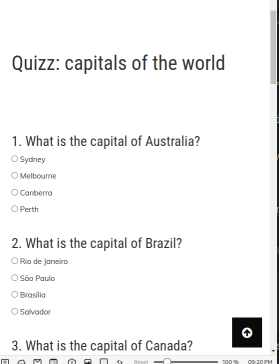Screenshot of an online quiz titled "QUIZZ: Capitals of the World" against a white background. A vertical scroll bar is present on the right side of the screen. The first question asks, "What is the capital of Australia?" with four multiple-choice options: Sydney, Melbourne, Canberra, and Perth. The second question follows, asking "What is the capital of Brazil?" with options: Rio de Janeiro, Sao Paulo, Brasilia, and Salvador. The third question pertains to the capital of Canada, but the full question is obscured and partially cut off. At the bottom of the browser, a row of icons is visible alongside a magnifying slider for zooming in or out on the webpage. The current time is displayed at 9:20 p.m. on the bottom right corner of the screen. Additionally, a black box featuring an up arrow is located in the bottom right corner of the webpage itself. The questions and answer options are listed with bubbles next to each choice, and there is a notable gap between the quiz title and the first question.